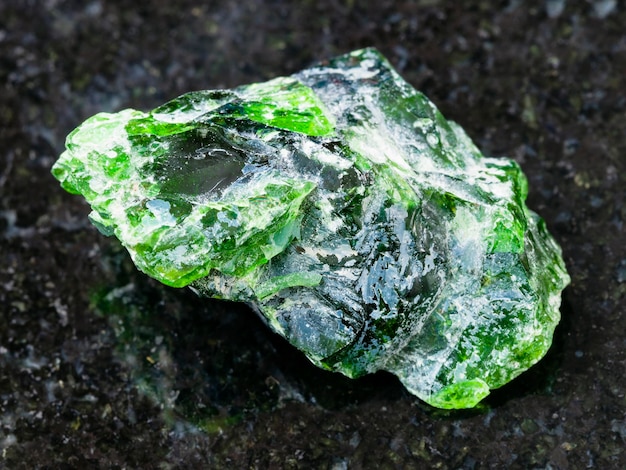The image showcases a striking, translucent green object, prominently positioned at the center and occupying nearly the entire frame. This object, which might be a jagged shard of green glass or a rough-hewn stone, exhibits a captivating mix of dark and light green hues, with some areas appearing almost white. The texture is rugged, with sharp angles and rough surfaces, suggesting it may have been recently unearthed. The object reflects light in a shiny, glassy manner, enhancing its translucent quality. It lies on a gritty, possibly dirt or gravel surface, and the high level of zoom and focus makes it seem nearly tangible. The background includes other green flecks and dark brown or black elements, hinting at a natural, outdoor setting where similar stones or shards might be found.